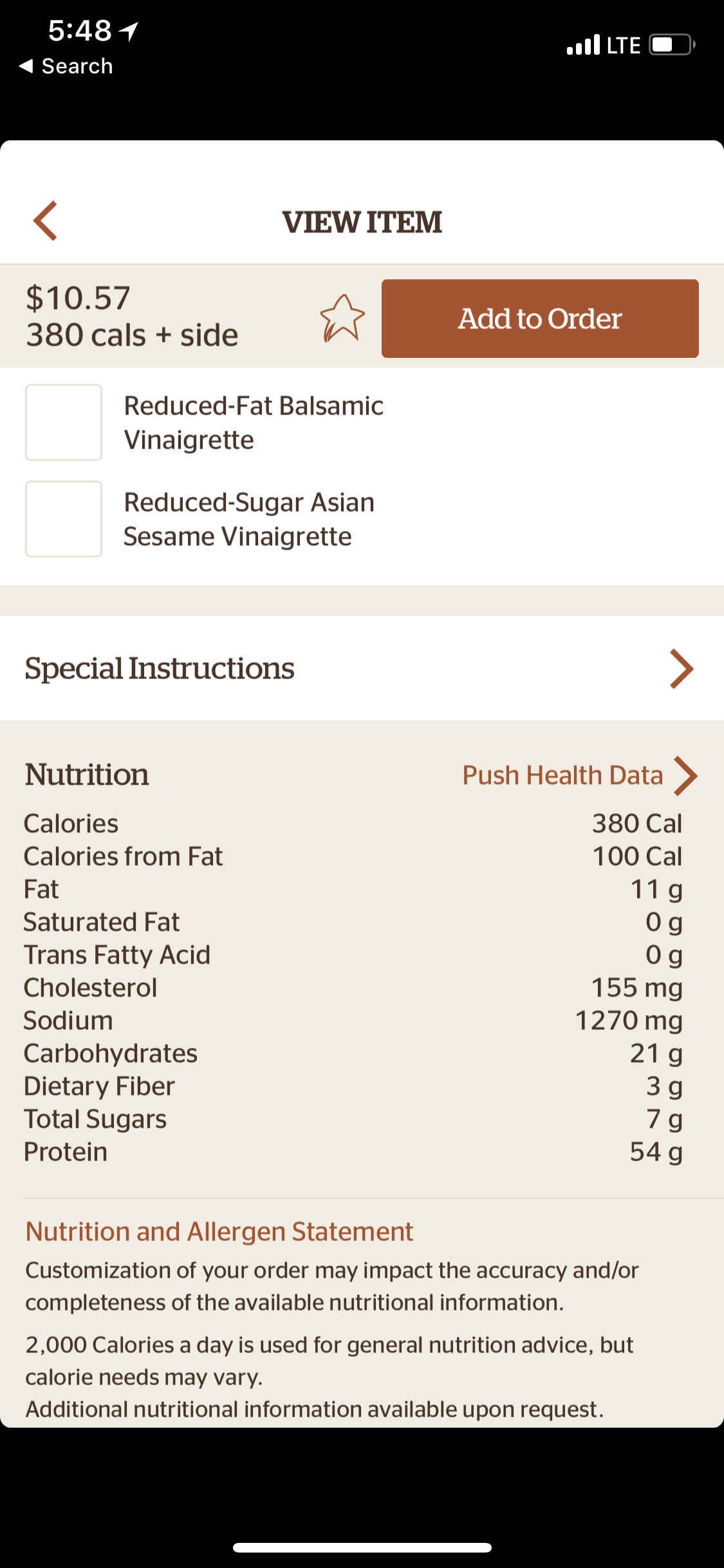This image is a screenshot of an order summary. At the top of the screenshot, there's a black rectangle containing the time "5:48" displayed in the upper left corner. To the right of the time, there are indicators for cell service bars, the "LTE" network status in white, and the battery charge level, also in white.

The background beneath this black bar is white. Centrally located is the phrase "View Item" in black text. Directly to the left of this text is a beige rectangle showing the price "$10.57". Below this price, there is the text "380 cows plus side."

To the right of the beige price box, there is a brown rectangle with the text "Add to Order" in white. Beneath these elements are two vinaigrette options, each bordered by faint, light brown squares. A thick, light gray line spans the width of the image separating these options from the section below.

Further down, there is a section for special instructions, indicated by the text "Special Instructions" positioned to the left against a white background. Directly below this section, there is a beige square containing nutritional information. At the very bottom of the image is a black rectangle.